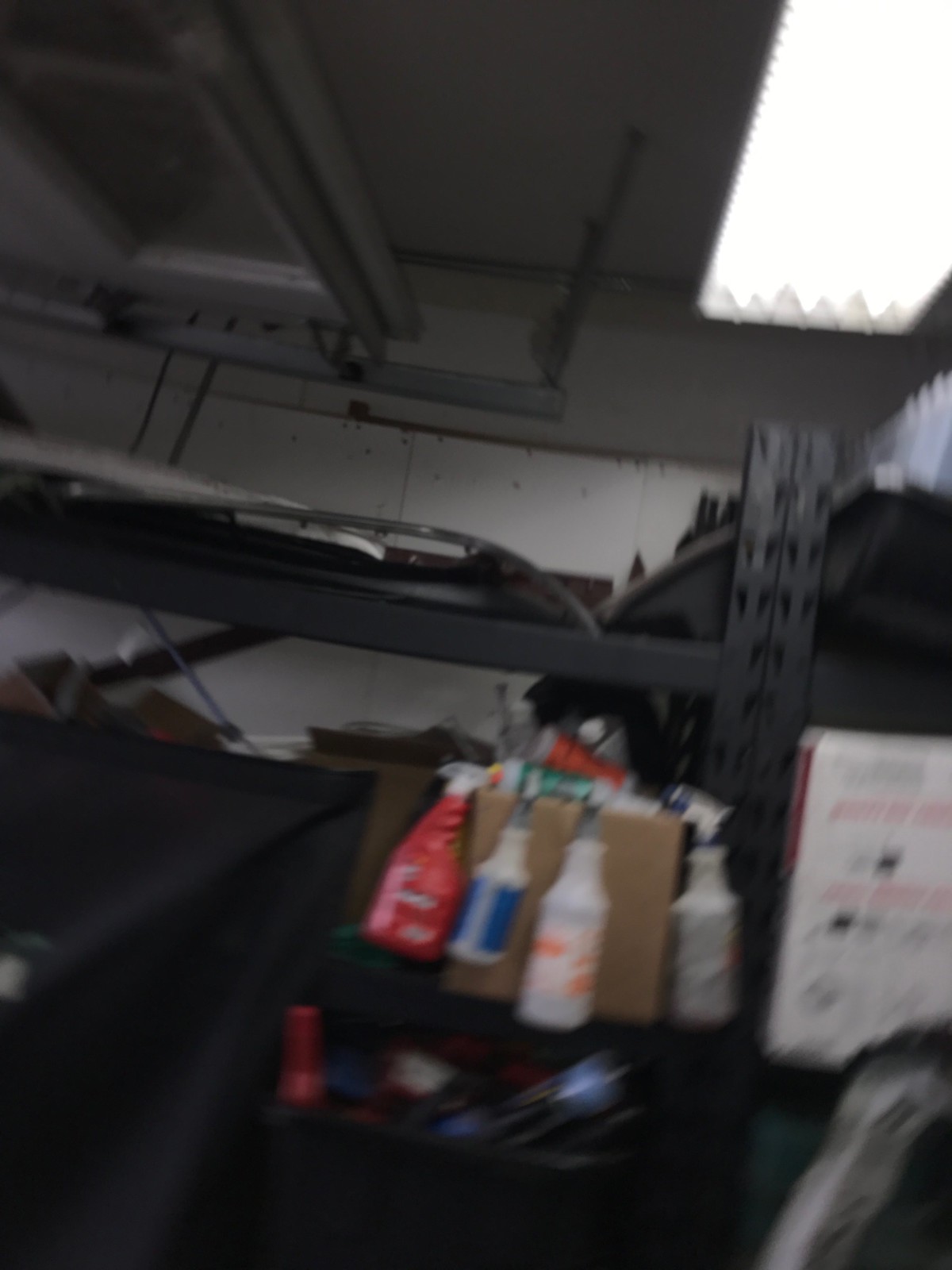The blurry photo appears to depict the interior of a dimly lit garage. The angle of the shot is from behind a large black metallic shelving unit, creating a cluttered scene. Numerous items are stored on the shelves, most notably a prominent brown cardboard box with several spray bottles hanging off its side—identified as a red bottle, a blue-labeled white bottle, and at least two more white bottles. Below this box sits a black bin containing an indistinct red-handled item and other miscellaneous blue objects. Adjacent to this, there is another white box positioned to the right in the image. A partially visible car, primarily white in color, is obscured by the shelf and various stored objects. There's an overhead fluorescent light fixture in the top right corner, while part of the garage door track and the door itself can be seen at the very top of the image, indicating that the garage door is open. The surrounding walls appear to be either white or pale gray, consistent with the typical setting of a home garage filled with assorted items, including what looks like tubing and other stored materials.